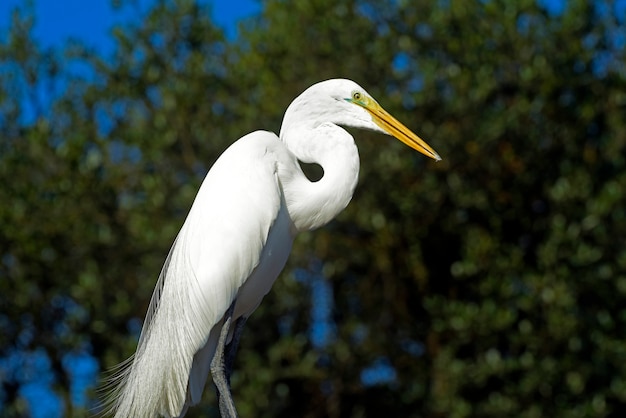The image captures a close-up profile of a heron, standing alone with its S-curved neck and head facing right. The heron is predominantly white, accentuated by wispy feathers being gently blown in the wind. It features a long yellow beak tinged with green around its small, beady eyes. The heron's legs are a striking charcoal gray, providing a sharp contrast to its pristine feathers. The background is artistically blurred, rendering a beautifully blended mix of a deep blue sky or water, coupled with verdant greenery and some trees, which emphasizes the bird's defined details against the muted colors. The high-quality focus on the heron highlights its graceful poise and the intricate textures of its plumage.